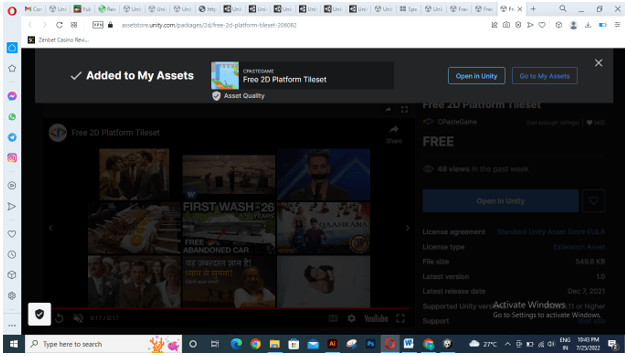The image depicts a webpage with a predominantly black background, creating a striking contrast with the illuminated interface elements. At the top of the screen, a header reads "Add to My Assets" and offers a "Free 20 Platform File Set." On the right side, two interactive buttons are visible: one highlighted with the text "Open in Unity" and a second, greyed-out button labeled "Go to My Accounts."

Behind the dark overlay of the webpage, faint images of various faces and objects appear, suggesting either magazine covers, film thumbnails, or other media, although the exact content is indiscernible. Bold white capital letters spell out "FREE" above a conspicuous blue box situated in the center of the screen. 

The webpage seems to be associated with Unity, as inferred from the interface and likely the URL entered by the users. Along the bottom edge of the computer screen, typical system icons are arranged, adding to the authenticity of a browser interface.